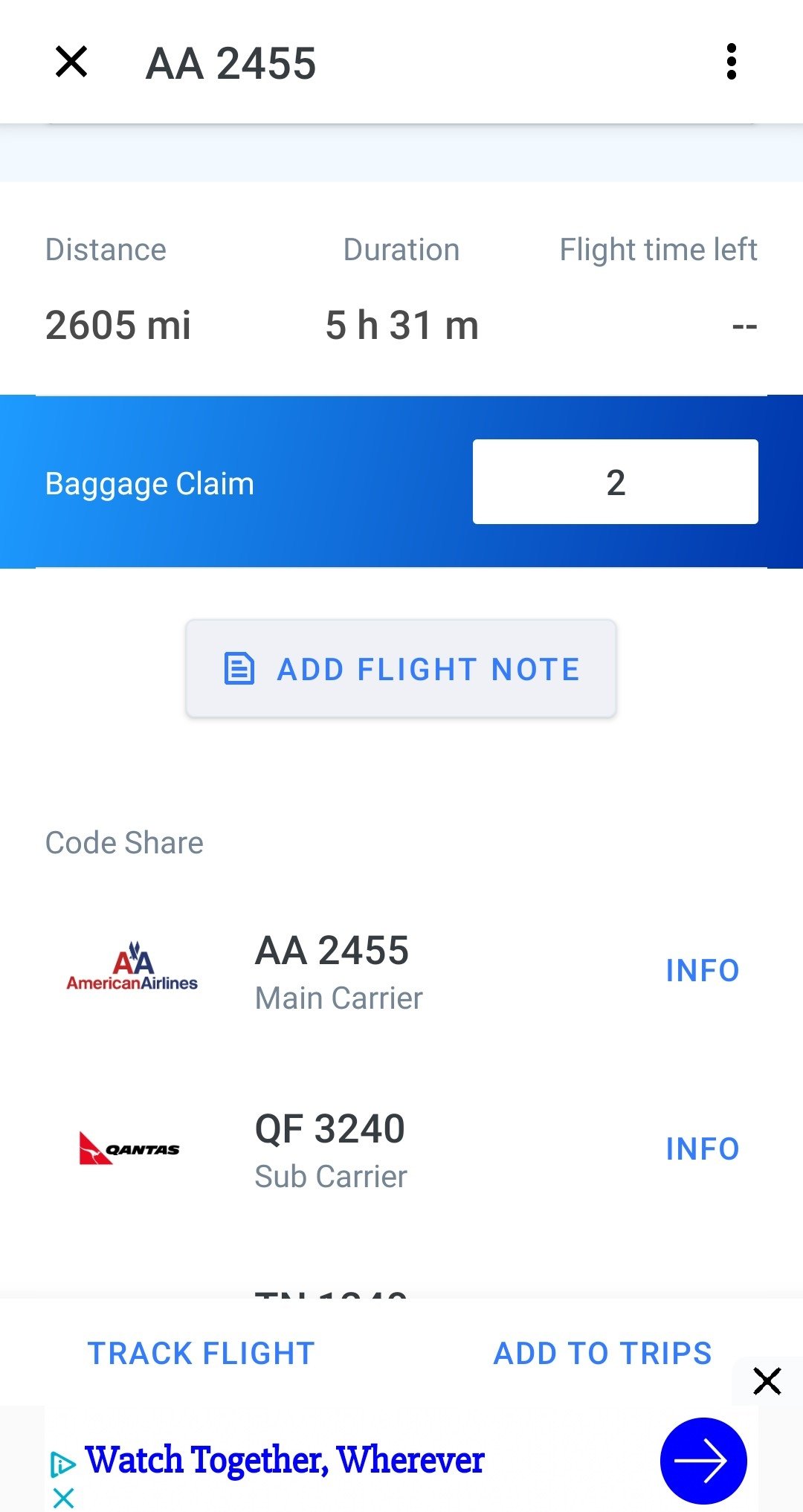Screenshot of a flight tracking application on a mobile device.

At the top, there's a retractable banner displaying the flight number "AA2455" and an 'X' button, suggesting that this banner can be closed. The upper right corner features a button with three dots, indicating additional options.

The app details the flight specifics:
- Distance: 2,605 miles
- Duration: 5 hours and 31 minutes
- Flight Time Left: Indicated with double dashes, signifying that the flight has ended.

Below this section, there is a blue rectangle labeled "Baggage claim" with the number "2" inside, indicating the baggage claim area. Following this is a gray button with blue text that reads "Add Flight Note," accompanied by a notepad icon.

Further down, the main airline carrier information is displayed:
- American Airlines (AA2455)
- Blue clickable button labeled "Info"

Underneath, there's another airline symbol for Qantas (QF3240) marked as the subcarrier, with a similar "Info" button.

The view is partially obscured by an ad and additional tabs at the bottom of the screen:
- Tabs: "Track Flight" and "Add Trips"
- Advertisement text: "Watch together wherever"
- A prominent blue arrow button in the bottom right corner.

This comprehensive list of elements provides a detailed overview of the flight's status as captured on a mobile flight tracking application.